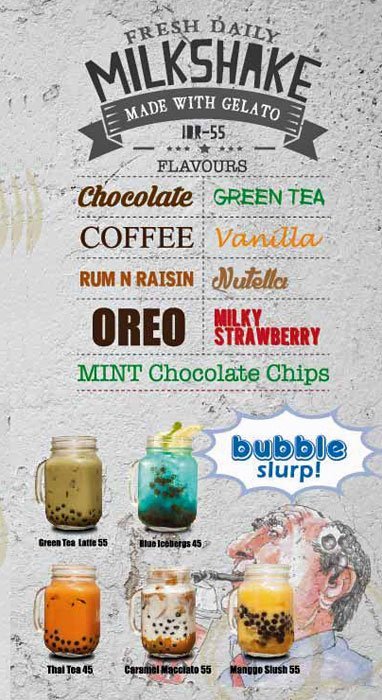The advertisement showcases a "Fresh Daily Milkshake Made with Gelato," available in a variety of flavors. The grayish background with black text lists an array of flavors in a neatly formatted table. The flavors and their respective colors are as follows: Chocolate (brown), Green Tea (green), Coffee (brown), Vanilla (light orange), Rum and Raisin (light brown), Nutella (light brown), Oreo (dark brown), Milky Strawberry (red), and Mint Chocolate Chips (mint green). At the bottom, five vibrant drinks are displayed in mason jars with handles, each containing brown bubbles indicative of bubble tea. The flavors of these drinks are Green Tea Latte ($5), Blue Iceberg ($5), Thai Tea ($4.50), Caramel Macchiato ($5), and Mango Slush ($5). Each drink is distinct in color: brown, blue, orange, white and brown, and orangish-yellow respectively. A cartoonish drawing of a man in the background enthusiastically drinking one of the beverages adds a playful touch to the advert, which is further emphasized by the "Bubble Slurp" text in blue lettering.